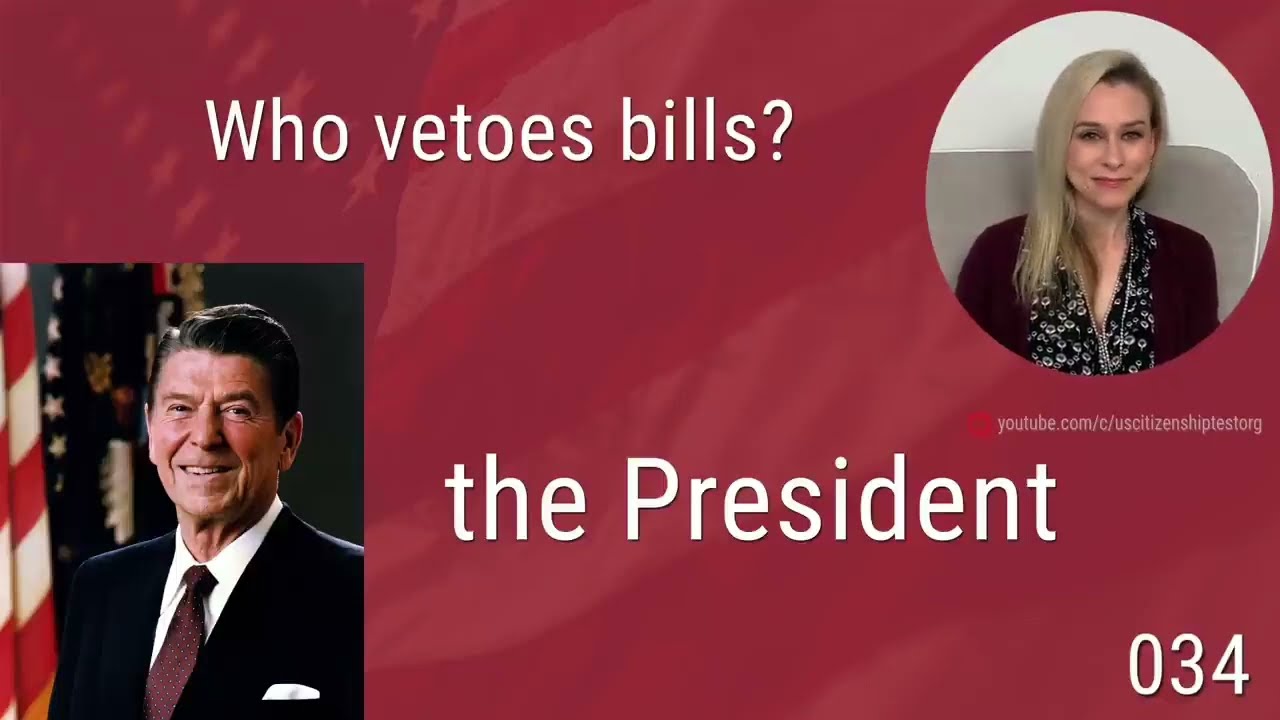The image appears to be a slide from a slideshow or a screenshot from a video on the internet, possibly from a webpage on YouTube at the URL "youtube.com/uscitizenshiptest.org." The background features the American flag with a red overlay. At the top of the image, in white letters, it asks, "Who vetoes bills?" Located at the top right is a partially visible image of a woman with long blonde hair, wearing a black and white floral shirt. Below her, it states "The President" in white letters. On the bottom left, there is an image of Ronald Reagan, smiling and dressed in a black jacket and a burgundy tie. In the bottom right corner, the number "034" is displayed in white.